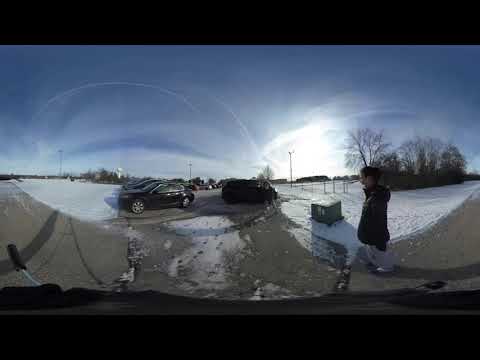In a wintry landscape characterized by a clear blue sky and wispy clouds, a man in a black coat and gray pants stands facing left on a snow-dusted sidewalk. To his right, an expansive snow-covered lawn hosts a large green electrical box. The scene unfolds with a parking lot full of cars to the left, extending down the center of a converging road. The area is lined with barren trees devoid of leaves, reflecting the cold season. In the background, a distant water tower and buildings are faintly visible. The sun is rising towards the center-right of the scene, casting a soft glow on the snow and highlighting the crisp, white expanse that surrounds the scene.